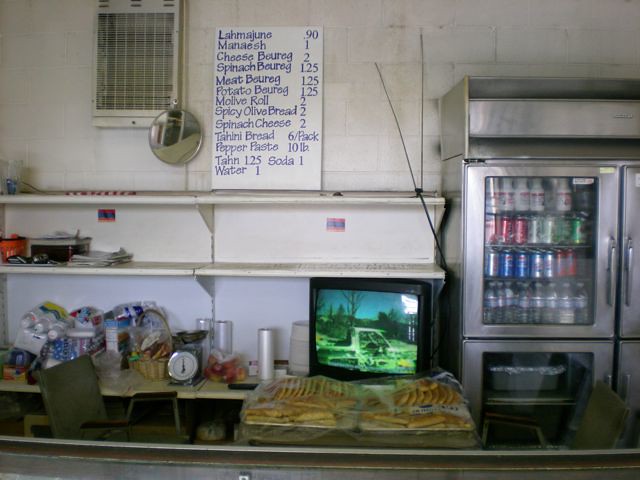The image depicts a small, outdoor food stand with a rustic vibe. At the back of the stand, there is a cinder block wall, suggesting the possibility of a compact kitchen or a walk-up café within. To the left of the stand, white shelves are crowded with a miscellany of items including a TV, plastic containers, lids, and a scale. Disposable cups are also stacked among the clutter. Adjacent to the shelves stands a four-door refrigerator, stocked with cans of soda, cartons of milk, and various food items arranged at the bottom.

On the back wall of the stand, a mirror reflects part of the bustling scene. Accompanying the mirror is a sign listing various food items and their prices: Amajun - 90 cents, Maneesh - $1, Cheese Boreg - $2, Spinach Boreg - $1.25, Meat Boreg - $1.25, Potato - $1.25, Olive Roll - $2, Spicy Olive Bread - $2, Spinach Cheese - $2, Tahini Bread (6 pack) - $6, Popper Pasta - £10, Tying - $1.25, Soda - $1, and Water - $1. Each element of the stand blends to create a picturesque and functional eatery, inviting customers to stop by and savor the variety of affordable, tantalizing offerings.